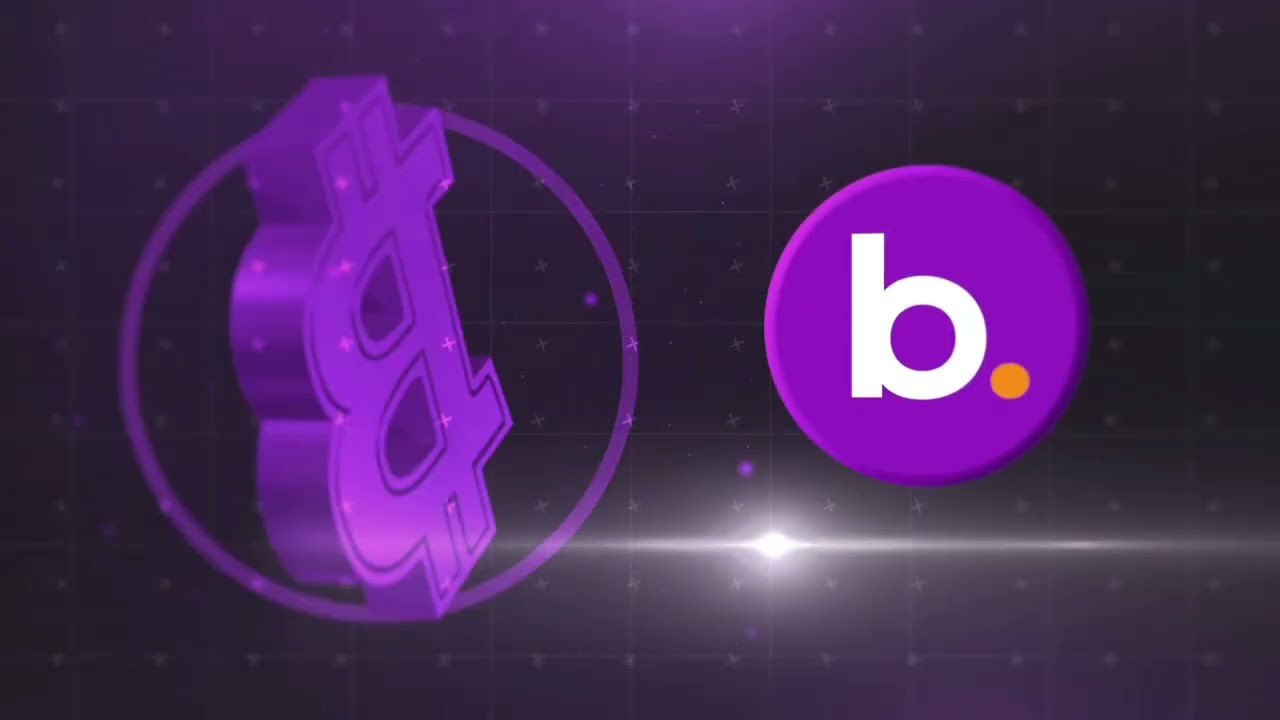The image is a graphic design featuring two logos against a dark purple backdrop. On the left side, within a purple-outlined circle, is the Bitcoin logo. This logo is an upside-down, tilted, and mirrored capital "B" with dollar sign strikes at the top and bottom, depicted in purple. Behind the logo, a grid pattern with blurred, small X's, suggesting stars at each vertex, is visible. To the right of the Bitcoin logo, a second circular logo appears with a lowercase "b" in white, followed by a period in light orange at its bottom right. Both logos are set against a background that transitions into a blurred black grid pattern with a bright white horizontal light beam extending from the bottom center beneath the lowercase "b" logo, radiating outwards.